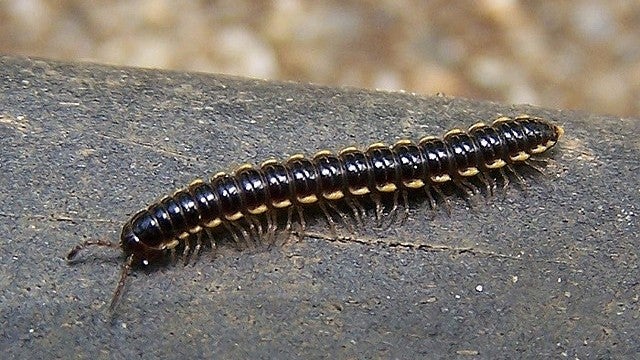This professionally captured close-up image showcases a long, black centipede in striking detail, with a yellowish-white line running along each side of its segmented body, which ends in a similarly colored tail. Its many spindly legs are visibly splayed along its length. The centipede's two prominent antennae protrude from its head, placed in the lower left corner of the image. The creature rests on a surface that appears to be a stone or brick, exhibiting a predominantly gray color with white spots, while some brown hues are also present. The blurred background, indicative of an outdoor setting, reveals a subtle pattern of swirled brown and white tones, adding to the natural ambiance of the photograph.